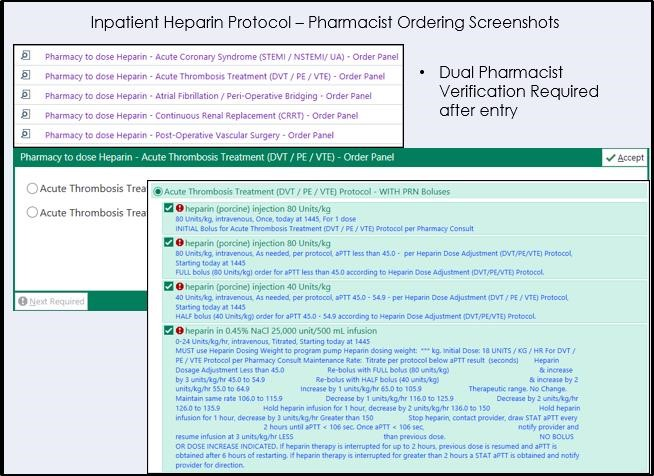**Caption:**

A screenshot from a medical website illustrating the Inpatient Heparin Protocol for pharmacists ordering screens. The main headline reads, "Inpatient Heparin Protocol Pharmacists Ordering Screenshots." There are two stacked screenshots, with one partially visible behind the other, resembling a presentation slide.

The background screenshot displays a list of order panels with several options: 
1. "Pharmacy to Dose Heparin - Acute Coronary Syndrome"
2. "Pharmacy to Dose Heparin - Acute Thrombosis Treatment"
3. "Pharmacy to Dose Heparin - Atrial Fibrillation"
4. "Pharmacy to Dose Heparin - Continuous Renal Replacement"
5. "Pharmacy to Dose Heparin - Postoperative Vascular Surgery"

The option "Acute Thrombosis Treatment" is selected with a checkbox next to it. To the right, there is a bullet point stating, "Dual Pharmacist Verification Required After Entry." Below, a subtab titled "Acute Thrombosis Treatment" contains additional checkboxes and detailed information relevant to the treatment protocol.